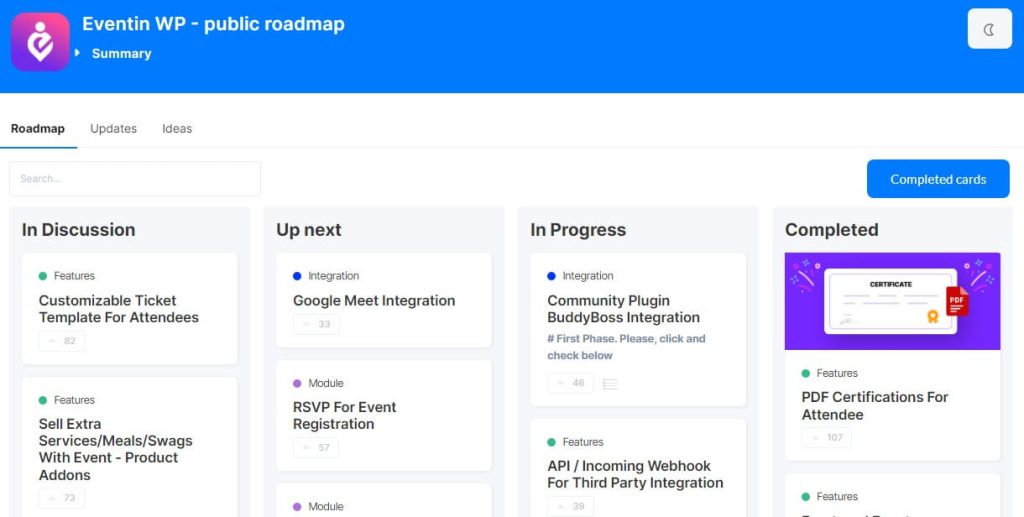This screenshot captures a web page from the Eventin WP Public Roadmap. The page features a dark blue banner at the top displaying the text "Eventin WP Public Roadmap: Summary." Below the banner is a navigation menu with options: Roadmap (selected), Updates, Ideas, Search, and Completed Cards.

The main content starts with sections labeled as "In Discussion," "Up Next," "In Progress," and "Completed." 

In the "In Discussion" section, there are plans for a "Customizable Ticket Template for Attendees," alongside features like "Sell Extra Services/Meals/Swags with Event Product Add-ons."

The "Up Next" section lists forthcoming integrations and modules such as "Google Meet Integration" and "RSVP for Event Registration," though the text for the latter is partially cut off.

In the "In Progress" section, it highlights "Community Plug-in" and "Buddy Boss Integration," with a note to "please click and check below." This section also features "API/Incoming Webhook for Third-Party Integration."

The "Completed" section showcases a visual representation of a certificate within a purple rectangle. The certificate features black text, gray lines mimicking writing, and a gold ribbon at the bottom right corner. Sparkly icons adorn the top left and right edges of the certificate, accompanying the feature's description of "PDF Certifications for Attendee." Sadly, the description is cut off at the bottom edge.

This detailed roadmap offers users insights into past, present, and future enhancements of the Eventin WP platform.